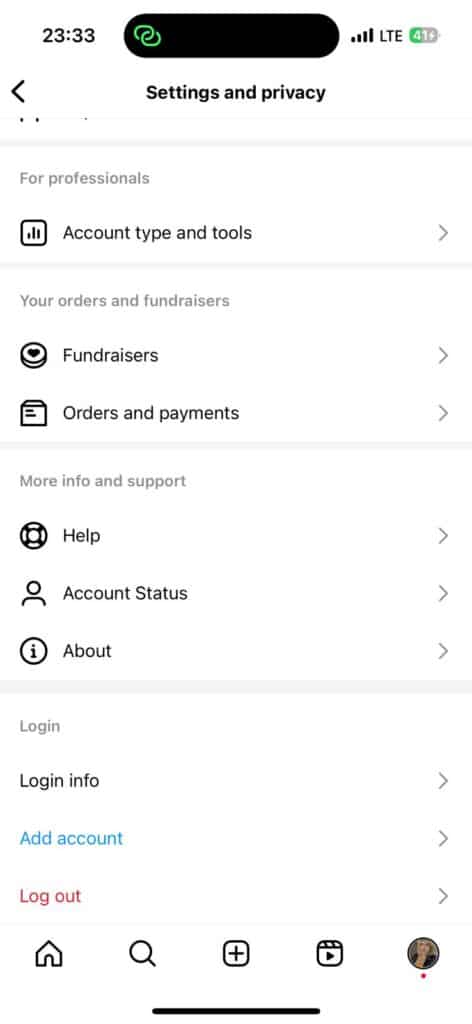The screenshot depicts a section of a mobile phone's user interface with a predominantly white background. At the top left corner, the time is displayed in bold black military format. Central to this upper section, there is a black oval icon, with two linked ovals situated to its left. On the right side, the reception and battery indicators are visible. Directly below this, in bold black text, the words "Settings" and "Privacy" are centered.

On the left edge below the title, there's a backward-pointing black arrow, resembling a sideways "V", indicating the back function. Beneath this arrow, there's a light gray horizontal line. Following this, the phrase "For Professionals" appears in gray text on the left. 

Two lines below, there is an icon on the left side accompanied by the text "Account Type and Tools" in black, with a gray right-pointing arrow (sideways "V") on the right side. A light gray line separates this from the next section, where the gray text reads "Your Orders and Fundraisers."

This category features two rows:
1. The first row has an icon on the left and the word "Fundraisers" in black, with a gray right-pointing arrow on the right.
2. The second row also starts with an icon on the left, followed by the phrase "Orders and Payments" in black, along with the gray right-pointing arrow on the right.

Another light gray horizontal line separates this section from the "Mobile Support" section which includes three lines:
- "Help"
- "Account Status"
- "About"

Each is listed in gray text.

Yet another gray horizontal line is below this, splitting it from the final section labeled "Login." Under this label:
- "Login Information" appears in black.
- "Add Account" is highlighted in blue.
- "Log Out" is marked in red.

All three options feature a right-pointing arrow on the right side of their respective lines.